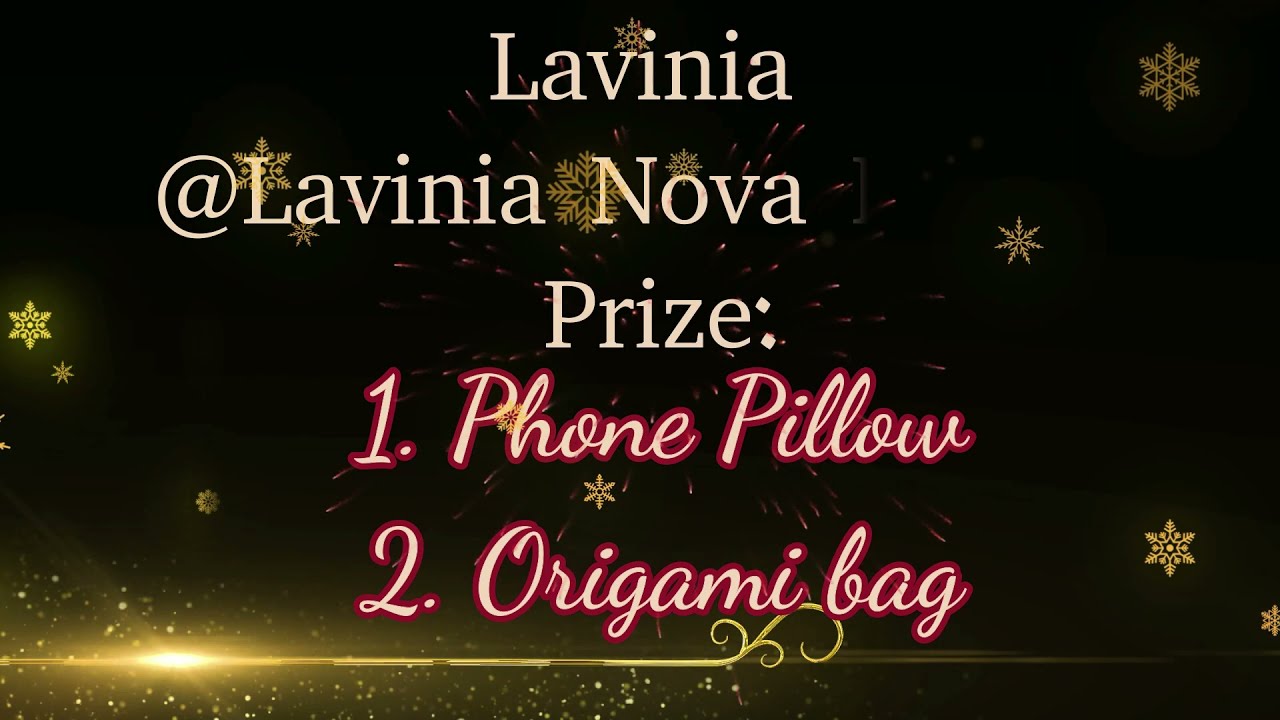The image is a visually striking advertisement poster with a predominantly black background adorned with scattered gold snowflakes. The design includes a prominent, reflective gold banner spanning the bottom of the image, ending in a scroll-like flourish. At the heart of the poster, central text in various colors and fonts reads:

"LaVinia at LaVinia Nova  
Prize:  
1. Phone Pillow  
2. Origami Bag"

The text at the top, "LaVinia at LaVinia Nova," is rendered in tan letters, while "Prize:" is white. The items "Phone Pillow" and "Origami Bag" are displayed in an electric script alternating between pink and blue-pink hues. Throughout the background, additional gold snowflakes sprinkle the imagery, with a notable gold snowflake positioned bottom right and another smaller one on the left edge. Hints of red and white accents are also speckled across the design, enhancing the festive appearance. Overall, this poster exudes a celebratory and elegant ambiance, likely designed for a special event or giveaway.